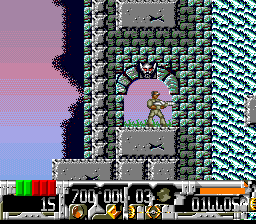In this detailed screenshot from a video game, the scene is set against a gradient sky that transitions from light blue at the horizon to a deep purple at the top. Dominating the scene is a turquoise building resembling a castle, constructed from greenish bricks. The focal point is an arched doorway, decorated with a menacing silver skull with glowing red eyes at its apex. A character clad in a light green outfit stands in this doorway, holding a silver gun and looking to his left while seemingly prepared to shoot. This character stands on a metallic, rectangular block, which is supported by two smaller blocks underneath and flanked by a large block on the left side. The bottom part of the screen displays the HUD, showing an assortment of game indicators and statistics like a health bar and various numbers: 15, 700, 000, 03, and possibly 014405, all encased in metal framing indicative of game settings and status.